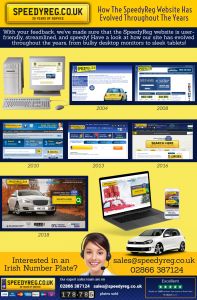A screenshot of the Speedy Reg website showcases its evolution over the years, adopting a striking yellow and blue color scheme. At the top, on a yellow background, a headline highlights the transformation of the Speedy Reg website. Below this, a small black-bordered yellow button is prominently labeled “speedyreg.co.uk.” 

Directly beneath the button, a blue banner features a message indicating that user feedback has driven the website's redesign to be more user-friendly, streamlined, and efficient. The banner invites viewers to explore the site's evolution, from outdated bulky desktop monitors to modern, sleek tablets. 

A visual timeline illustrates this progression with various icons: starting with an old white desktop computer, moving through a more sophisticated black flat-screen from 2004, and advancing to laptops, tablets, and smartphones, reflecting the technological advancements over the years. 

At the bottom of the screenshot, an inquiry about Irish number plates is presented. A woman with brown hair, wearing a headset, is depicted alongside contact information: “sales@speedyreg.co.uk” and the phone number “02866 387 124.” Above her, an image of a white car adds a visual cue to the service being offered.